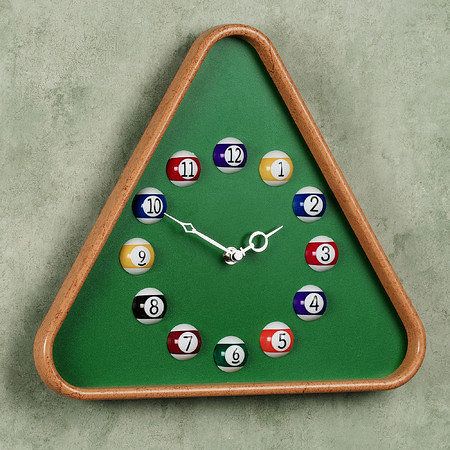This detailed photograph features a unique wall clock mounted against a marbled cream background with dark gray and light gray blotches. The clock is shaped like a billiards rack, characterized by its rounded triangular frame, resembling the wooden frame used to organize billiards balls. The clock face is light green, similar to the surface of a pool table. For the numbers, each hour marker is represented by a billiards ball, correlating with the actual colors and numbers found in a billiards set. The balls range from 1 to 12: the 1 and 9 are yellow, the 2 and 10 are blue, the 3 and 11 are red, the 4 and 12 are purple, the 5 is orange, the 6 is green, the 7 is dark red, and the 8 is black. The center of the clock is metallic, with the small hand currently pointing at 2 and the long hand at 10.